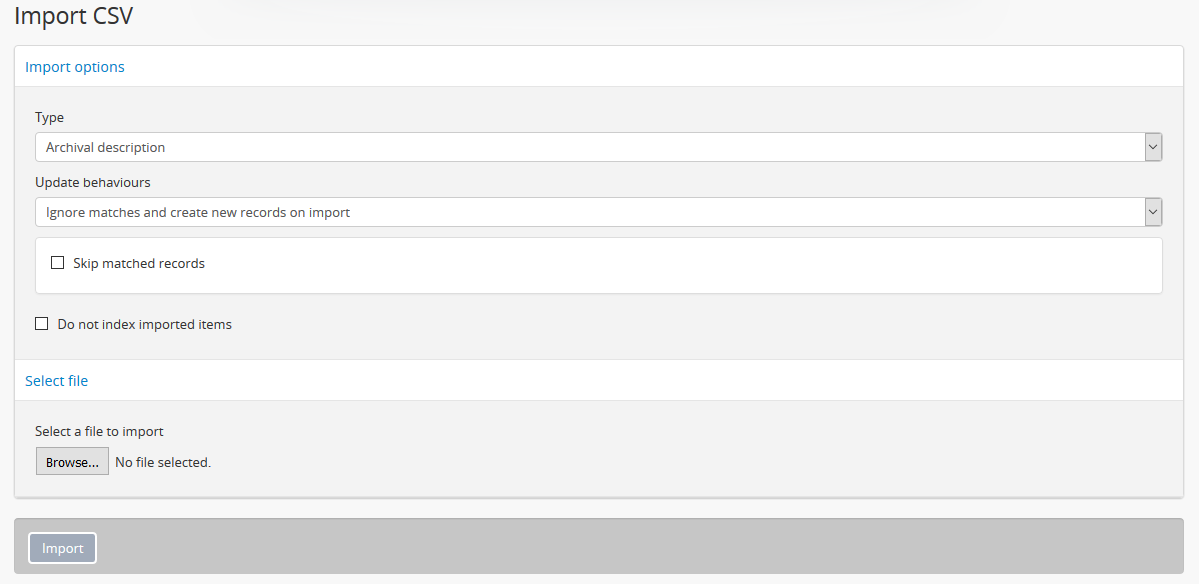The interface displays various options for importing a CSV file into the system. The top section features a gray line with the label "Import CSV." Underneath, on a white bar, the text "Import Options" is highlighted in blue. Below this, within a gray background, there's a section titled "Type," and in the corresponding data space, "Archival Description" is indicated in gray on a white bar. Following that, another section labeled "Update Behaviors" appears, detailing the action "Ignore matches and create new records on import" within a white data bar. 

Beneath this section, another white bar presents the option "Skip matched records" accompanied by an unchecked checkbox. Similarly, the option "Do not index imported items" is displayed with an unchecked checkbox. Further down, a white bar with the title "Select file" is shown in blue, prompting the user to select a file to import. Adjacent to this is a "Browse" button and a notification that states "No file selected."

At the bottom of the interface, a gray bar includes the "Import" button, which stands out in white text with a white outline against a brownish-gray background. Overall, the interface is designed to facilitate the importation of CSV files with clear and organized options.